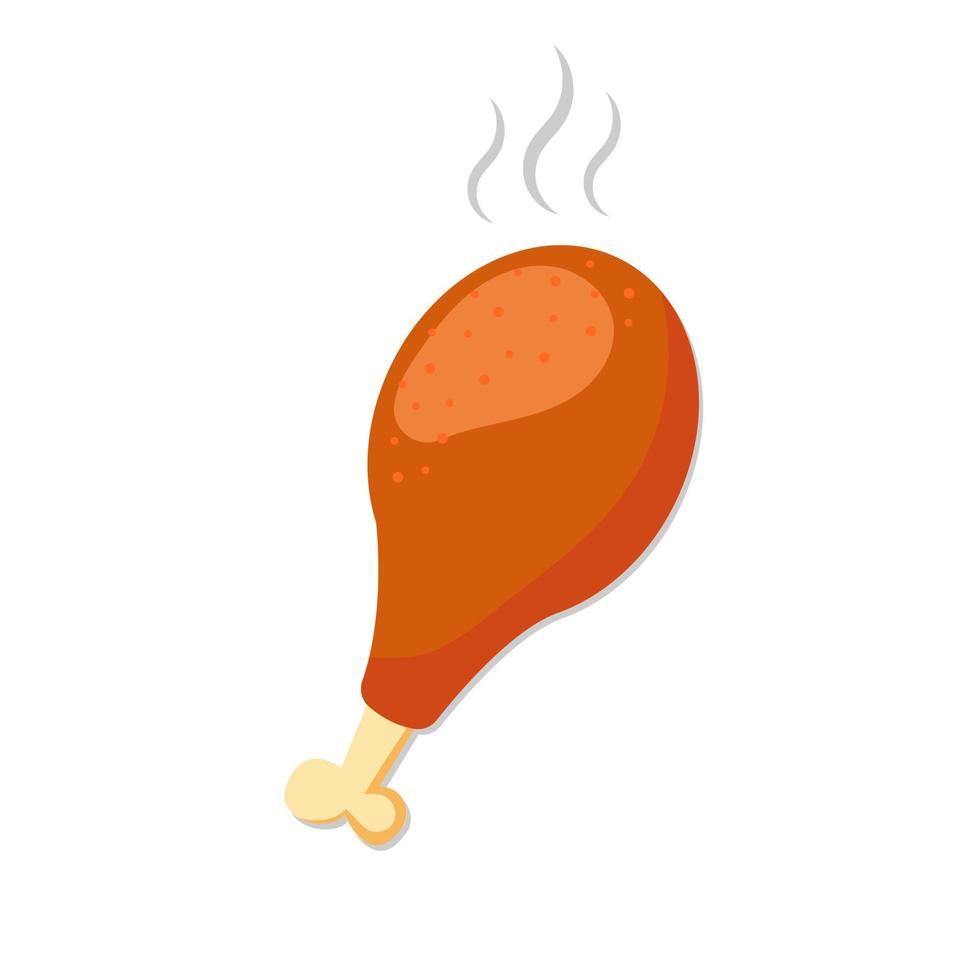The image is a graphic representation, rendered in a clip art style, of a drumstick that appears to be from either a chicken or turkey. Set against a solid white background, the drumstick is pointed bone-side down with the exposed bone positioned at the bottom left-hand side of the image. The bone is a light tan or cream color, transitioning to the flesh part which is a reddish-brown or dark brown shade. The top portion of the drumstick features a lighter brown or pinkish oval shape, dotted with similarly colored contrasting dots. Above the drumstick, there are three wavy gray lines, suggesting that the meat is steaming hot. The overall aesthetic is simplistic and exaggerated, reminiscent of a primitive or cartoonish style, much like something one might see in a Flintstones episode, emphasizing its stylized and non-realistic nature.